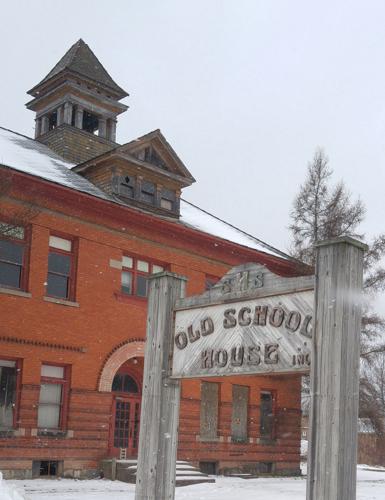In the image, a red-bricked school building with gray tiles and a distinctive tower rises against a snowy winter backdrop. The front features an arched entrance and red doors, with snow covering the steps leading up to it. Prominently displayed in the foreground is a weathered gray wooden sign with raised letters, reading "Old School House, Inc. SHS." The wood on the sign varies in tone, with the "Old School House" part appearing lighter, almost white, and the "Inc." section in a darker shade. The building is framed by leafless trees, and the sky above is completely white, suggesting an overcast, wintry day. Snow blankets the ground and the roof, emphasizing the chilly atmosphere.